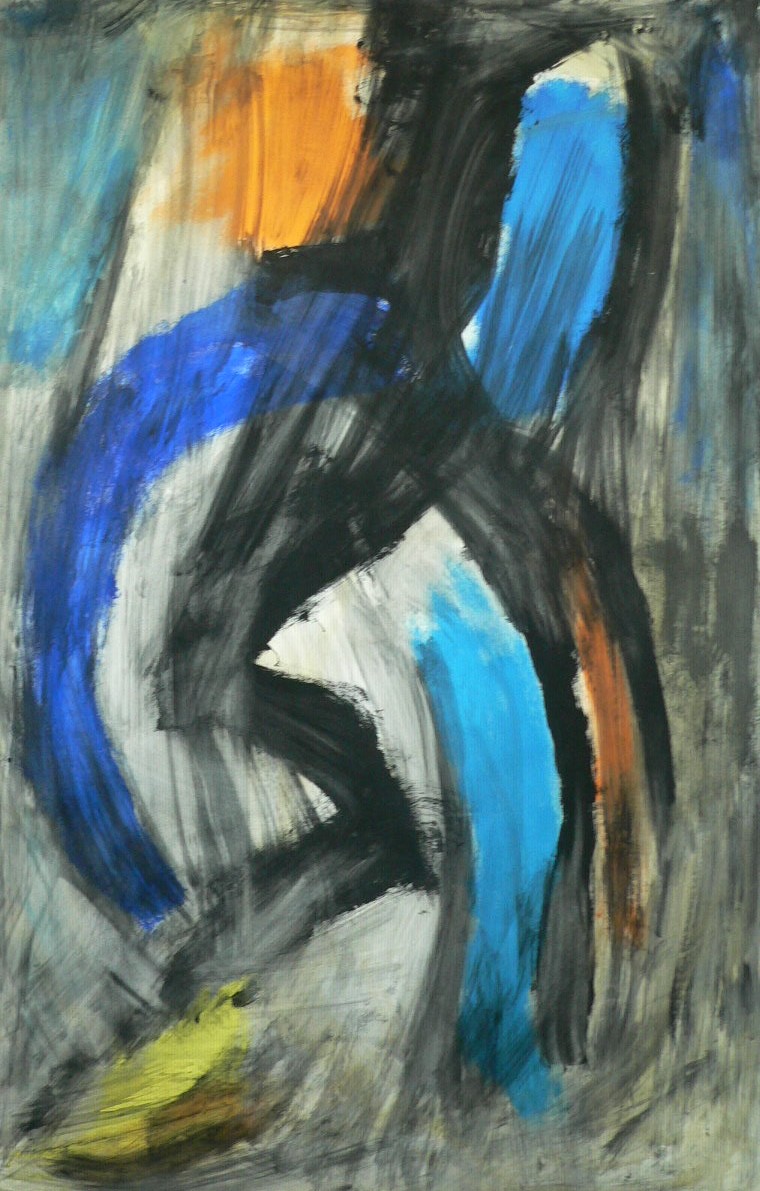This abstract watercolor painting features an intricate composition of colors and shapes. At the center of the image is a prominent black structure resembling a lightning bolt or zigzagging line that begins at the upper right corner and extends down the page. This black line splits into three sections: one curving downward to the right, another continuing straight with a sharp zigzag near the bottom, and a third segment that curves back to the left, ending in a yellow area at the bottom left of the image.

The background is a harmonious blend of light blue, dark blue, gray, and touches of orange, giving it a watercolor texture. In the upper left, blue and gray dominate, transitioning to white with a bit of orange as you move right, and then shifting to black across the top. This thicker black line thins out as it extends down the right side of the image.

In the middle left section, a blue semicircle begins at the black structure and curves to the left before slightly returning to the middle. The bottom left portion of the painting is mainly gray with the notable yellow part beneath the black form and intersecting blue curve. The bottom right corner features predominantly gray shades with hints of black.

Overall, the painting’s abstract nature and varied use of color and line create a dynamic and textured composition.